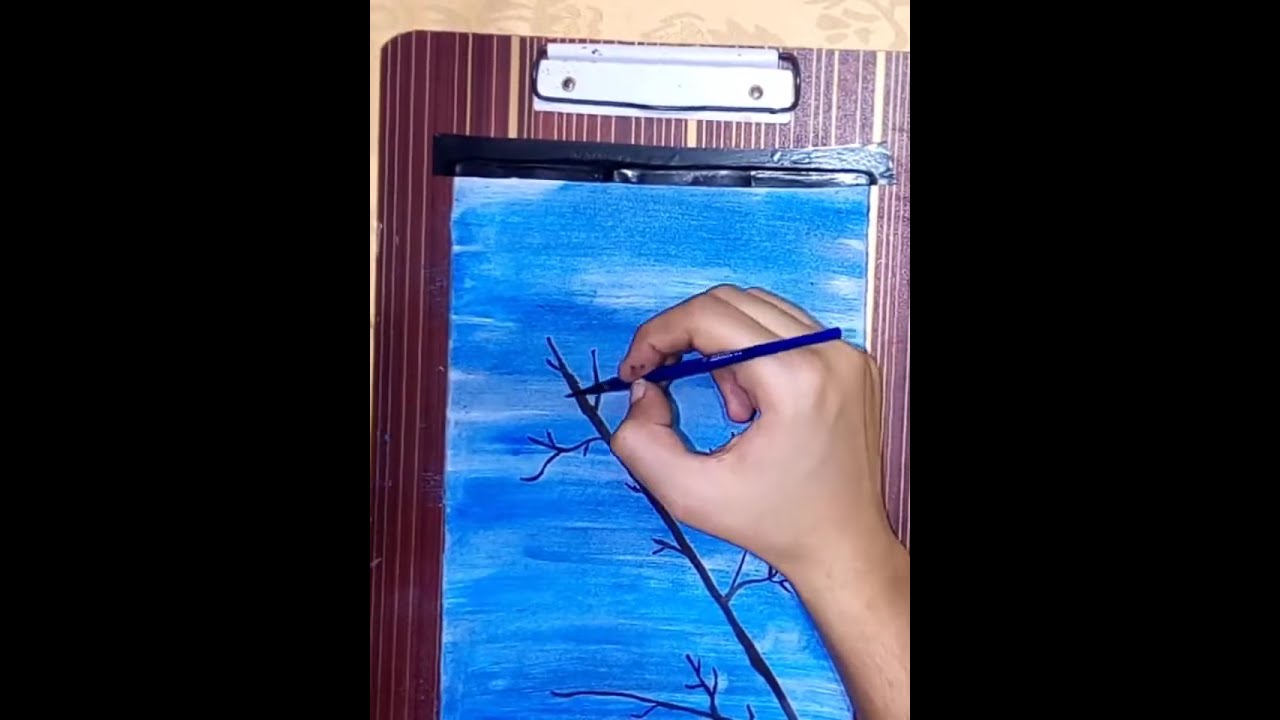The image depicts a detailed scene of an individual’s right hand, captured from the wrist to fingertips, as they meticulously draw a tree with branching limbs using a blue pen. The drawing is set against a bright blue background on a piece of paper that is adorned with a watercolor wash of varying shades of blue. Some areas of the background remain white, adding visual contrast. The paper is secured with black tape to a clipboard, featuring a rich purple or maroon hue with vertical beige or light brown stripes and a silver clip. The clipboard rests on a surface with a dark beige, swirling floral pattern. The scene suggests an artistic process, possibly a student or hobbyist working diligently at a desk or table, focusing intently on the intricacies of the drawn tree, which notably lacks leaves, resembling a bare winter tree.